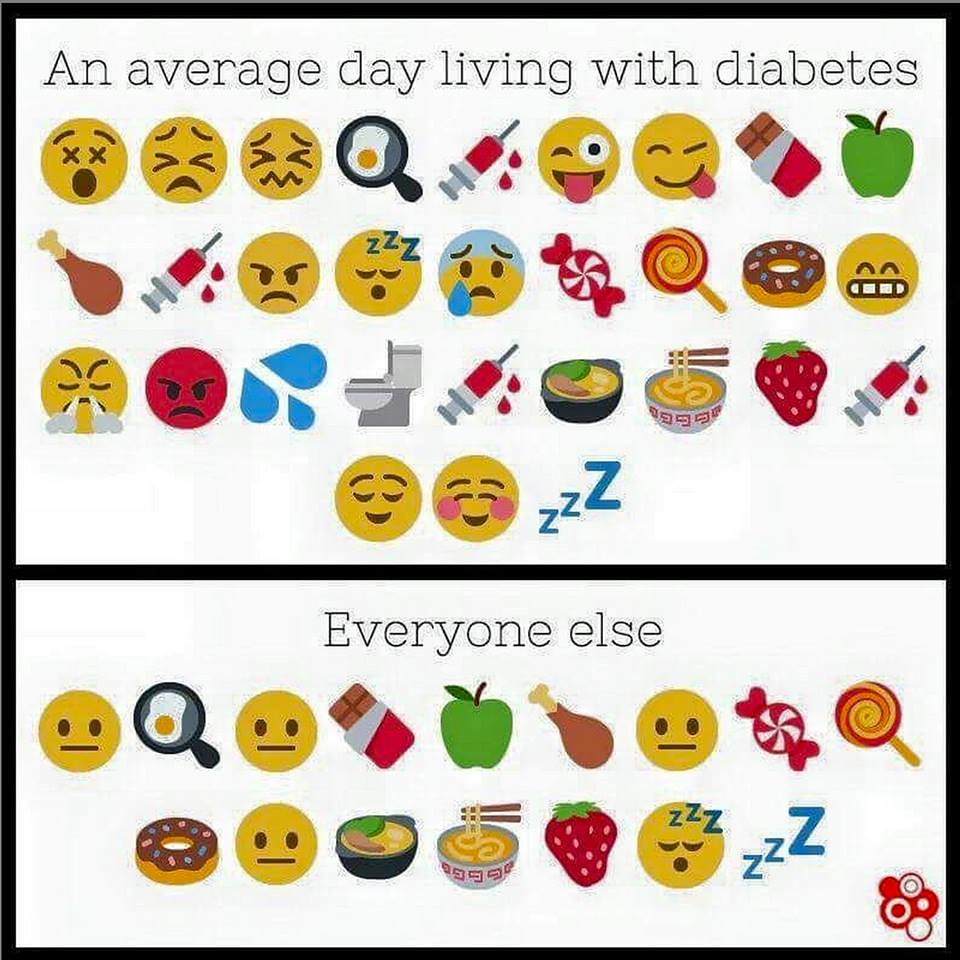The image is divided into two horizontal rectangular panels, with the larger panel at the top labeled "An Average Day Living with Diabetes" in black letters. This top panel is crowded with a variety of emojis, each representing different aspects of living with diabetes. These include sad faces, angry faces, syringes, medicine, magnifying glasses, and emojis with tears, illustrating the emotional and physical challenges faced by individuals with diabetes.

In contrast, the smaller panel below is labeled "Everyone Else" and features fewer, more content-looking emojis. These emojis represent a range of normal, everyday foods and emotions, including donuts, strawberries, apples, lollipops, candy, and happy or neutral faces, indicating a more stable and carefree lifestyle compared to those living with diabetes. The image starkly contrasts the chaotic and often distressing experiences of diabetics with the more balanced and less emotionally turbulent lives of non-diabetics.